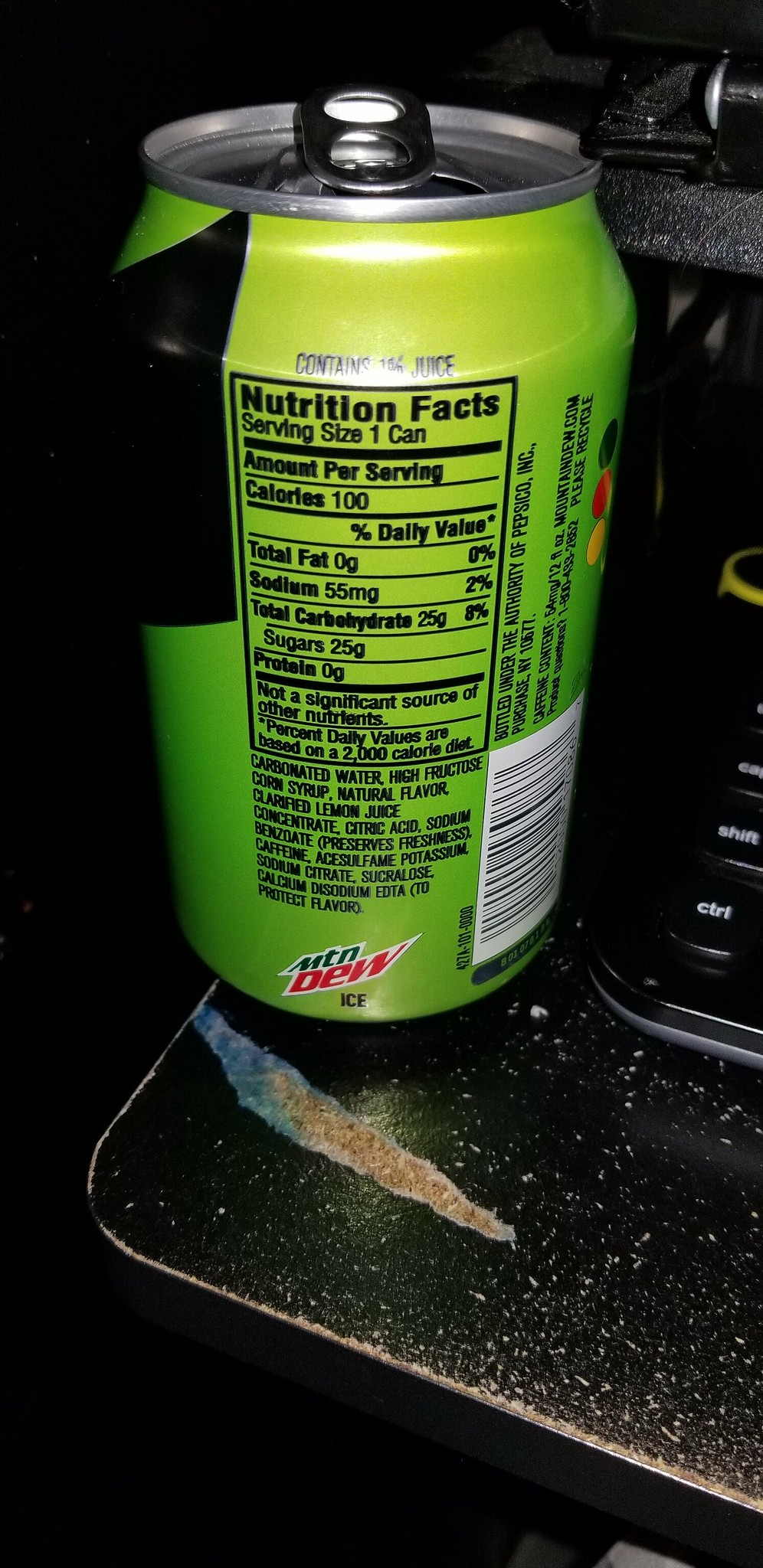A close-up image features the nutrition panel of a Mountain Dew Ice can, showcasing stylized "MTN DEW ICE" lettering in dark green, white, and red hues on a neon to light yellow-green gradient background. The can, which has been opened, details 100 calories and 25 grams of sugar per serving, though the juice content, possibly 10%, is obscured by light reflection. To the right, a barcode and ingredient list are visible alongside circle marks, likely for color testing during printing. The can sits on a worn black desk with visible particle board material exposed through a significant gouge. A black keyboard is partially visible, specifically its control, shift, and caps lock keys. The scene suggests a gaming setup with a computer monitor likely perched on a second shelf in the background. There's a black and yellow object partially visible, adding contrast to the predominantly dark-colored setting.